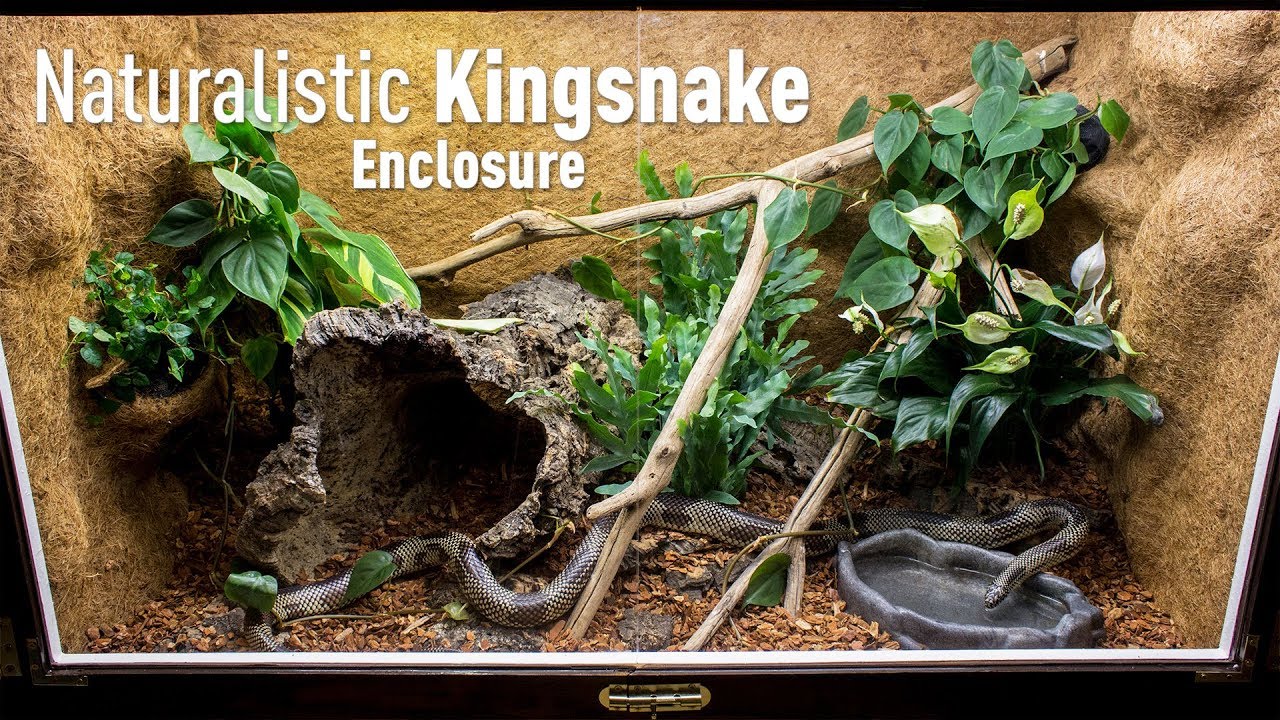The image depicts a detailed and naturalistic kingsnake enclosure within a glass terrarium, commonly used either for personal pets or reptile displays in zoos. The enclosure features a substrate that appears to be a mix of brown moss, coconut fiber, and rocks, creating a textured ground layer. Dominating the space are several broken tree branches adorned with green leaves, offering climbing opportunities and visual appeal, and a large, hollowed-out log situated towards the bottom left, serving as a cave-like retreat for the snake.

At the bottom right, there's a shallow, gray plastic water dish mimicking stone, from which the brown and yellow, black and gray spotted kingsnake is seen drinking. The snake is stretched out comfortably across the terrarium, showcasing its length and coloration. The overall setup, designed to mimic the snake’s natural habitat as closely as possible, is labeled with white text at the top left corner of the glass panel, reading "Naturalistic Kingsnake Enclosure." This text suggests the image could possibly serve as an advertisement or educational display for potential reptile owners.